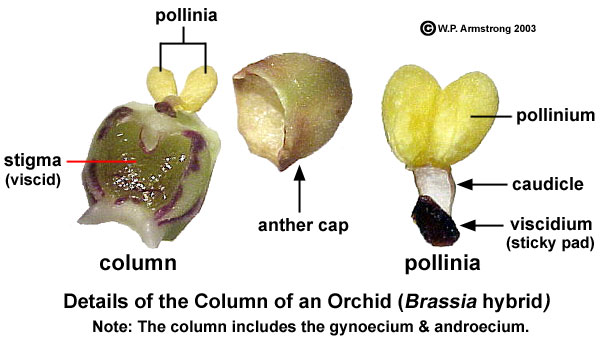This image features a scientifically detailed diagram of an orchid column, set against a white background, showcasing various dissected components of the plant, each meticulously labeled. Titled "Details of the Column of an Orchid" with the Latin name "Brassia Hybrid" in parentheses, the image provides an in-depth look at the flower's internal structure.

The diagram includes three primary photos of dissected orchid parts. From left to right:

1. The leftmost image, labeled "Column," highlights the stigma, with an added detail of the Pollenia situated atop the stigma.
2. The central image, labeled "Anthracap" (or potentially "Amphicamp" as referenced), depicts a green, gelatinous interior resembling the inside of a grape, adorned with white and purple exterior markings.
3. The rightmost image, labeled "Pollenia," provides a close-up view of the yellowish, puffy pods, illustrating intricate details such as the sticky pad (Pollenumum) and cortical structures.

In addition to these labeled parts, the diagram specifies auxiliary structures, including yellow pods at the top, a greenish-white cap adjacent to the right, and a white stalk with a black tip at the bottom. The bottom section of the image features black lettering, reading, "Note the column includes the Gynoseum and Androeseum," giving further insight into the detailed botanical anatomy presented.